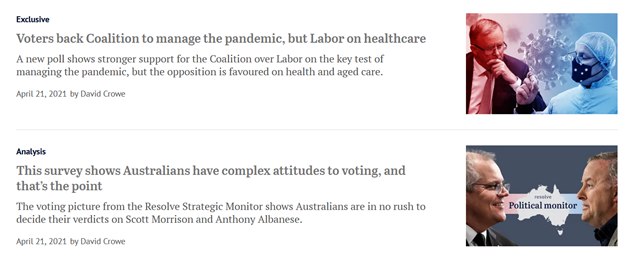Webpage Screenshot Featuring Two Articles

The screenshot captures a webpage listing two articles, each accompanied by an image and a brief description.

**Top Article:**
- **Headline:** "Exclusive: Voters Back Coalition to Manage the Pandemic but Labor on Health Care"
- **Photograph Description:** To the right of the headline, there's a digitally produced image. On the left side of this image, a man in a suit is depicted, while on the right side, a doctor wearing scrubs, a mask, and a head covering appears as though performing surgery. In the background, there's a digital representation of a virus cell.
- **Article Summary:** A new poll indicates that voters have stronger support for the coalition over Labor in managing the pandemic; however, Labor is favored when it comes to health and aged care.
- **Additional Information:** Date of publication is April 21, 2021. The article is authored by David Crowe.
- **Separator:** A faint line spans the width of the webpage, separating the two articles.

**Bottom Article:**
- **Headline:** "Analysis: This Survey Shows Australians Have Complex Attitudes to Voting, and That's the Point"
- **Photograph Description:** To the right of the headline, there is an image of two men facing each other; one is on the left side and the other on the right side of the photograph. In the background, the words "Political Monitor" are visible.
- **Article Summary:** The article delves into findings from the Resolve Strategic Monitor, revealing that Australians are in no rush to make decisive judgments on political figures Scott Morrison and Anthony Albanese.
- **Additional Information:** Date of publication is April 21, 2021. The article is also authored by David Crowe.